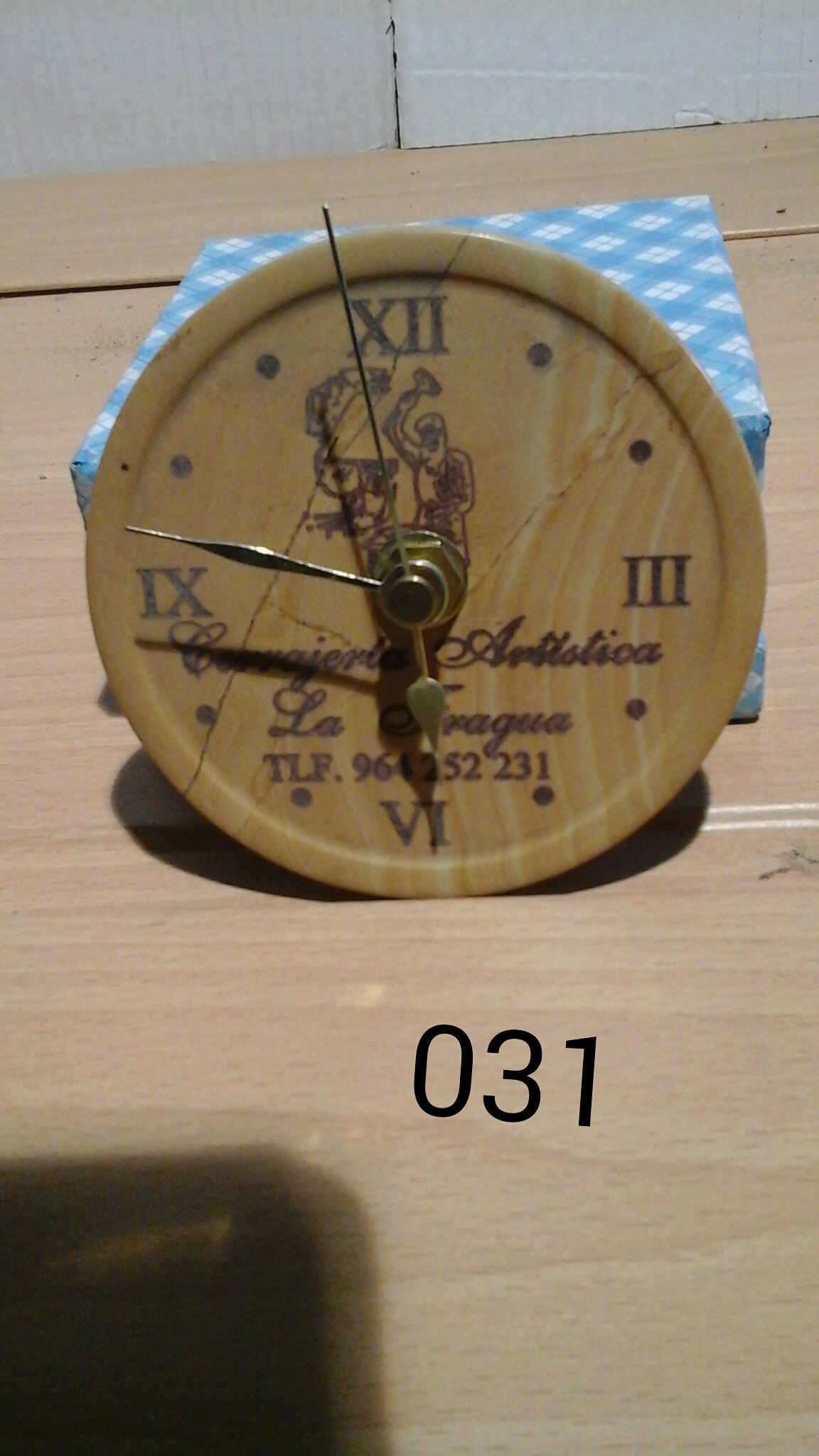The image showcases a detailed scene featuring a round, rustic clock with intricate details. The clock, made from what appears to be a solid piece of wood or possibly laser-etched wood, is positioned on a light wooden floor beside a white wall. It is propped up against a blue and white checkered box, resembling either a wrapped Christmas present or a decorative container. The clock itself displays Roman numerals for 12 (XII), 3 (III), 6 (VI), and 9 (IX), with simple dots marking the other hours. Standing out in brass or brass-colored metal are the hour and minute hands, poised just before 10:00, while an unusually long second hand extends well beyond the clock face. The face of the clock features an etched or engraved image of a blacksmith wielding a hammer, likely working at an anvil. Additional text on the clock includes "Artistica La Fragua," potentially in French, suggesting it may be an antique item. The bottom of the image also displays the watermark "031." Notably, the shadow of the photographer's phone is visible in the lower left corner, highlighting the casual, perhaps impromptu, nature of the photograph.